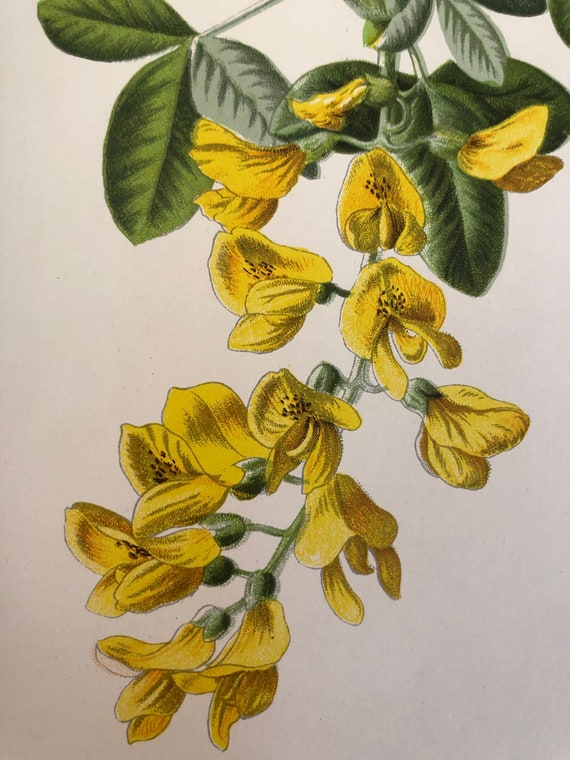This illustration features a delicate, hanging branch from what appears to be a tree or plant, set against a light pink backdrop. The top portion of the branch, approximately three to four inches, is adorned with green leaves. These leaves vary in appearance, ranging from standard green foliage to some with darker green stripes and a few showing a grayish tint. Below the leaves, the branch extends another 8 to 12 inches and hosts around 15 yellow flowers, somewhat resembling open daisy blossoms. Each flower emerges from a green, rugby ball-shaped bud, transitioning into yellow petals that house small, dark spots. The detailed rendering captures the natural beauty of the symmetrical arrangement and the subtle color variations, giving a lifelike quality to the charming botanical scene.